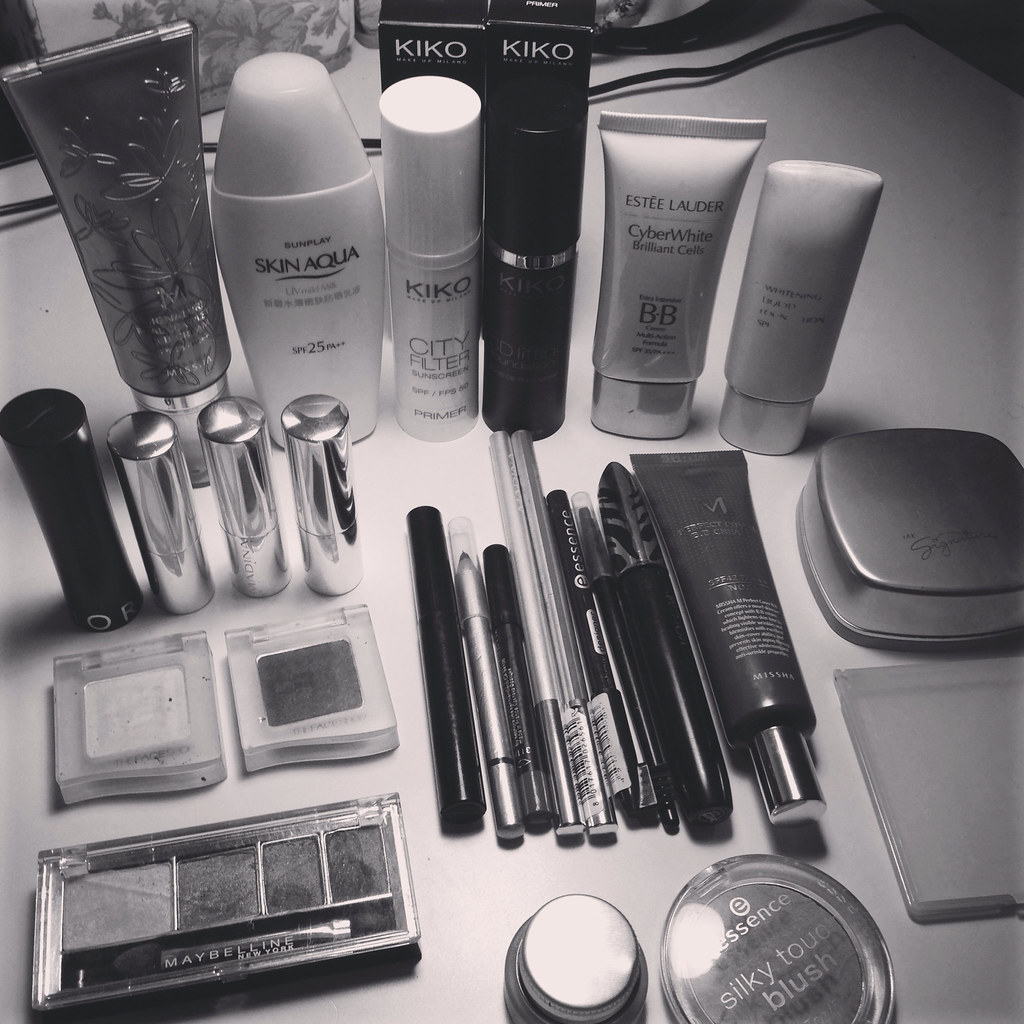The black and white photograph showcases a diverse array of makeup and skincare products spread out on a light-colored surface, possibly white or gray. The assortment includes various brands such as Skin Aqua, Kiko, City Filter, and Estee Lauder Cyber White. Specific items are also visible, including Essence Silky Touch Blush and Maybelline eye shadow. The collection features a variety of containers, including cylindrical lipstick tubes, eye shadow compacts, eyeliner, and blush cases, all with distinct shapes and sizes. The light source, positioned above the table, casts reflections on the glossy plastic lids and metallic lipstick cylinders, illuminating the scene with a soft, diffused glow. The myriad of brand names and product details inscribed on the containers adds to the intricate visual complexity of the composition.